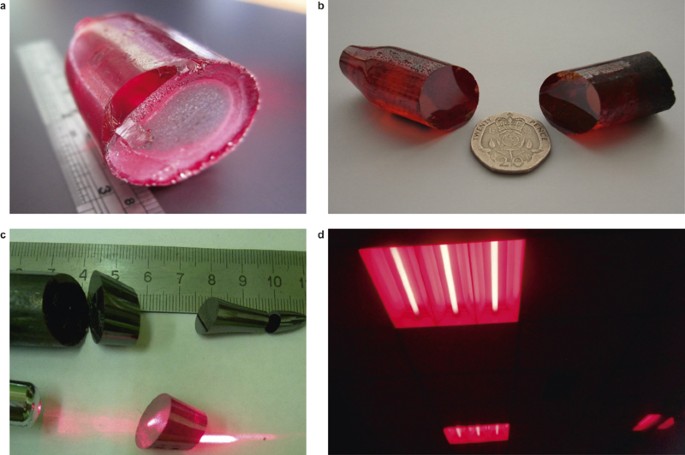The image consists of a 2x2 grid of photographs labeled A, B, C, and D, each showcasing various red gemstones, possibly rubies or similar crystals. 

In A, a single red, cut gemstone is shown next to a silver ruler on a silver surface, revealing its intricate facets and internal structure. 

Photograph B features two cherry-red, translucent gemstones flanking a gold coin with indistinct markings. 

Image C focuses on a ranging set of crystal and mineral fragments measured with a ruler. A distinctive cone-shaped red gemstone is illuminated by a thin light beam that creates a striking interplay of pink and yellow hues on the crystal. 

Lastly, D depicts an enigmatic array of trapezoidal red lights with overhead lighting against a black background, suggesting an artistic display or a creatively lit representation of the crystals. The consistency in the red hues across all photographs hints at the gemstones being the same or related materials.